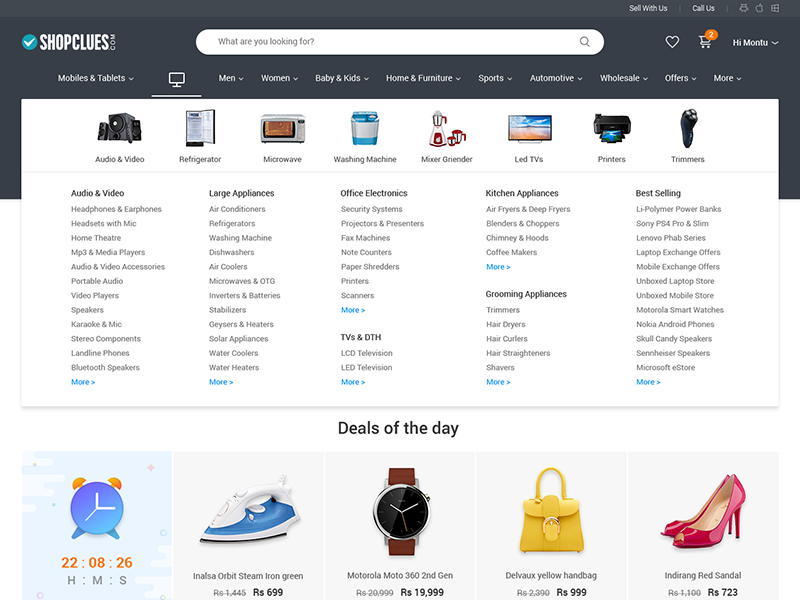**Detailed Caption:**

The image depicts a desktop screen displaying the homepage of an e-commerce website, ShopClues.

**Top Navigation Bar:**
- In the top left corner, there is a white check mark inside a blue circle, followed by the text "SHOPCLUES" in uppercase letters. Below "SHOPCLUES," the text "DOTCOM" is written vertically.
- To the right of the ShopClues logo, there is a long, white oval-shaped search bar. The phrase "What are you looking for?" is inside the search bar on the left, and a magnifying glass icon (search icon) is on the right.
- Beside the search bar, there is a heart-shaped icon, followed by a shopping cart icon. The cart icon has an orange circle with the number "2" in white within the circle, indicating two items in the cart.
- Further to the right, it says "HI MONTU" with a down arrow, indicating a dropdown menu. Above the heart icon, the text "SELL WITH US" is displayed.
- The text "CALL US" is placed above the shopping cart icon, separated by a vertical line from "SELL WITH US."
- Above "HI MONTU," there are three icons for different operating systems: Android, Apple, and Windows.

**Category Navigation Bar:**
- Directly beneath the ShopClues text, there are several categories listed horizontally: "MOBILES AND TABLETS" (with a down arrow), followed by "DESKTOP" (currently selected, indicated by an underline). Additional categories include MEN, WOMEN, BABY AND KIDS, HOME AND FURNITURE, SPORTS, AUTOMOTIVE, WHOLESALE, OFFERS, and MORE, each with a down arrow.

**Content Area:**
- Below the category navigation bar, the background changes from gray to white.
- The white box at the top features several category names with corresponding images. From left to right: AUDIO AND VIDEO (with an audio/video icon), SPEAKERS (with a speaker icon), REFRIGERATOR (with a fridge icon), MICROWAVE (with a microwave icon), WASHING MACHINE (with a washing machine icon), MIXER GRINDER (misspelled as "GRIENDER," with a blender and mixing bowls), LED TV (with a TV icon), PRINTERS (with a printer icon), and TRIMMERS (with a trimmer icon).

**Detailed Categories:**
- Below these icons, categories are organized into five columns, each featuring subcategories:
  1. **Audio and Video:** Headphones and Airphones, Headsets with Mic, Home Theater, MP3 and Media Players, Audio and Video Accessories, Portable Audio, Video Players, Karaoke Mic, Stereo Components, Landline Phones, Bluetooth Speakers, with "MORE" in blue and an arrow.
  2. **Large Appliances:** Air Conditioners, Refrigerators, Washing Machines, Dishwashers, Air Coolers, Microwaves and OTG, Inverters and Batteries, Stabilizers, Geysers and Heaters, Solar Appliances, Water Coolers, Water Heaters, with "MORE" in blue and an arrow.
  3. **Office Electronics:** Security System, Projectors and Presenters, Fax Machines, Note Counters, Paper Shredders, Printers, Scanners, with "MORE" in blue and an arrow.
  4. **TV and DTH:** LCD Television, LED Television, with "MORE" in blue and an arrow.
  5. **Kitchen Appliances:** Air Fryers and Deep Fryers, Blenders and Choppers (misspelled as "Vendors and Choppers"), Chimneys and Hoods, Coffee Makers, with "MORE" in blue and an arrow.
  6. **Grooming Appliances:** Trimmers, Hair Dryers, Hair Curlers, Hair Straighteners, Shavers, with "MORE" in blue and an arrow.
  7. **Best Selling Life:** Polymer Power Banks, Sony PS4 Pro and Slim, Lenovo, FOB Series, Laptop Exchange Offers, Mobile Exchange Offers, Unboxed Laptop Store, Unboxed Mobile Store, Motorola, Smartwatches, Nokia, Android Phones, Skullcandy Speakers (misspelled as "School Candy Speakers"), Sennheiser Speakers (misspelled as "Shenizer Speakers"), Microsoft E-store, with "MORE" in blue and an arrow.

**Deals of the Day:**
- At the bottom, there's a "DEALS OF THE DAY" section in the middle with a countdown timer showing "22:08:26" (H:M:S).
- Four grey background boxes showcasing various deals:
  1. An "INSTALLA ORBIT STEAM IRON GREEN" for Rs 1,445 discounted to Rs 699.
  2. A "MOTOROLA MOTO 360 SECOND GEN" smartwatch for Rs 20,999 discounted to Rs 19,999.
  3. A "DELLA VOICE YELLOW HANDBAG" for Rs 2,390 discounted to Rs 999.
  4. A pair of red high heels, "INDERON RED SANDAL" for Rs 1,100 discounted to Rs 723.